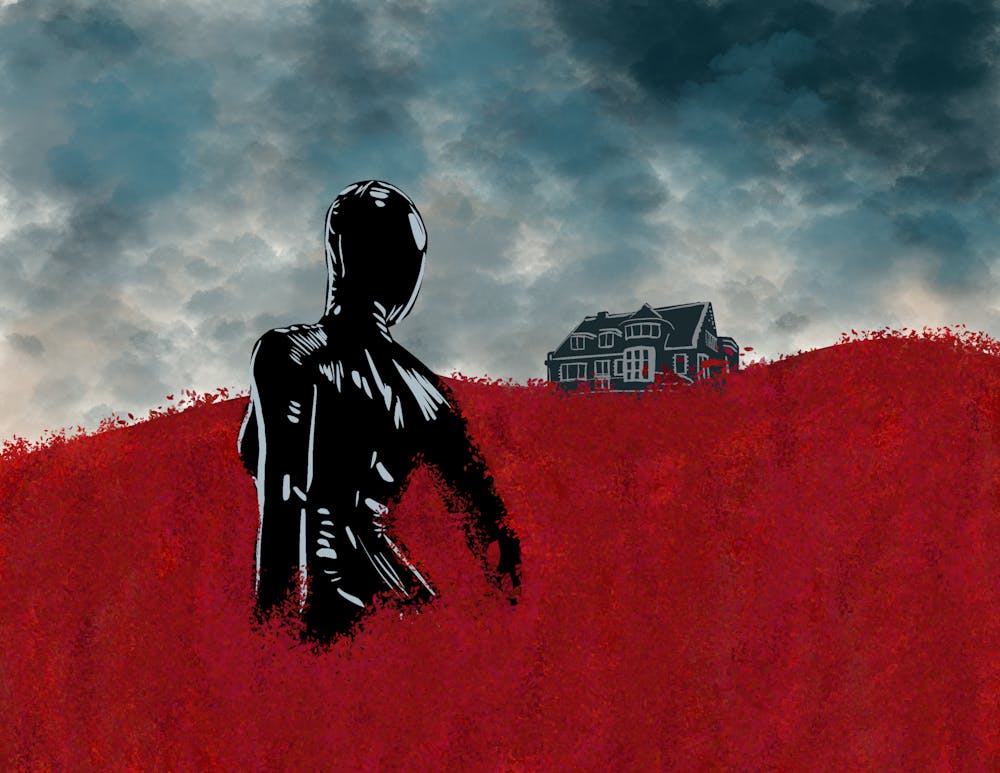The painting depicts a dramatic and ominous scene of a tall, turret-adorned house perched atop a blood-red hill, framed by a stormy and moody sky. The house, navy blue with white windows, stands in stark contrast against the backdrop of thick, dark clouds that range from deep blue to lighter hues, creating a menacing atmosphere. Below the house, a woman dressed entirely in black with white accent dots stands in a striking, almost statuesque pose within the waist-high, crimson foliage, which resembles tall weeds or grass. She has her back partially turned, with her head twisted over her shoulder to gaze at the distant house. Her form-fitting, almost cellophane-like attire accentuates her feminine silhouette, lending an even more surreal quality to the scene. The visual interplay between the vivid red field, the dark and stormy sky, and the starkly contrasting house and figure creates an eerie and captivating image.